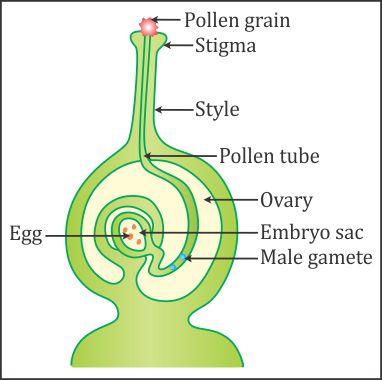This image is a detailed square graphic illustration on a white background, depicting the reproductive anatomy of a flower. The central focus of the image is a green structure with a long stem, labeled with various parts and accompanied by arrows for clarity. At the top, there is a bright pink dot labeled "pollen grain," which sits on the "stigma," the receptive tip of the green structure. Adjacent to it, the "style," a narrow neck-like channel, guides the pollen grain through the "pollen tube," highlighted within the stem. The illustration further points to the "ovary," which houses the “embryo sac” and "egg" in its middle, where fertilization takes place. Also labeled within this intricate system is the "male gamete." The image meticulously explains the journey of pollen from its initial contact on the stigma, down through the style and pollen tube, ultimately reaching the ovary to fertilize the egg, emphasizing the process of plant reproduction.